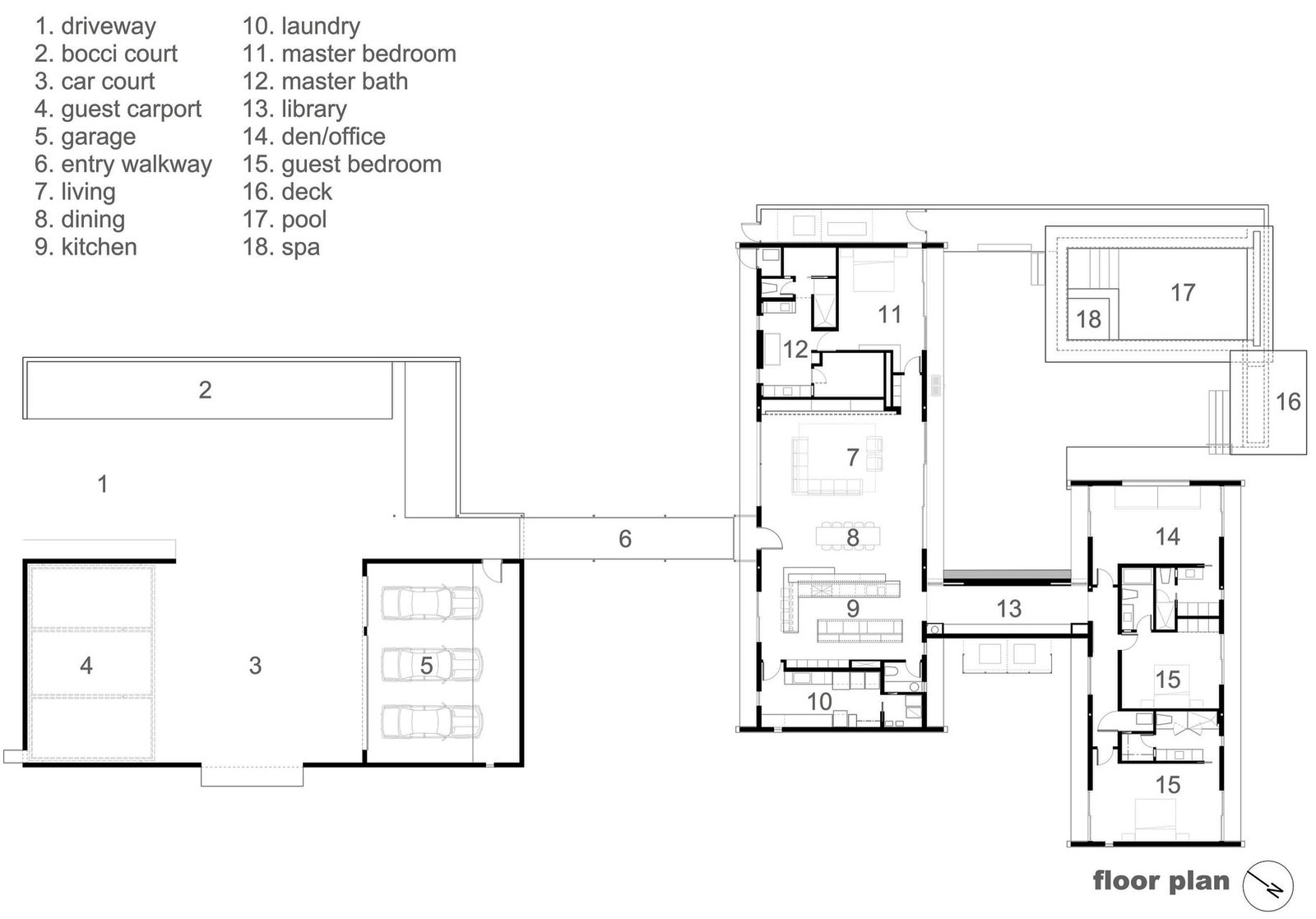The image is a simple black and white floor plan, reminiscent of what you might find online while searching for an apartment or house. The diagram is organized with numbered sections from 1 to 18, each corresponding to a specific area within the layout. At the top left, there is a key split into two columns: the first column lists numbers 1 through 9 and the second column lists 10 through 18. Each number is labeled to indicate different features and rooms: 1 is the driveway, 2 is the bocce court, 3 is the car court, 4 is the guest carport, 5 is the garage, 6 is the entry walkway, 7 is the living room, 8 is the dining room, 9 is the kitchen, 10 is the laundry, 11 is the master bedroom, 12 is the master bath, 13 is the library, 14 is the den/office, 15 is the guest bedroom, 16 is the deck, 17 is the pool, and 18 is the spa. The schematic shows the arrangement of these areas from an aerial perspective, with the layout divided into a left section including mostly outdoor and entry spaces, and a right section that comprises the main interior of the building. At the bottom right-hand corner of the image, the words "floor plan" are written in black letters, accompanied by an emblem indicating north at a 10 o'clock direction.